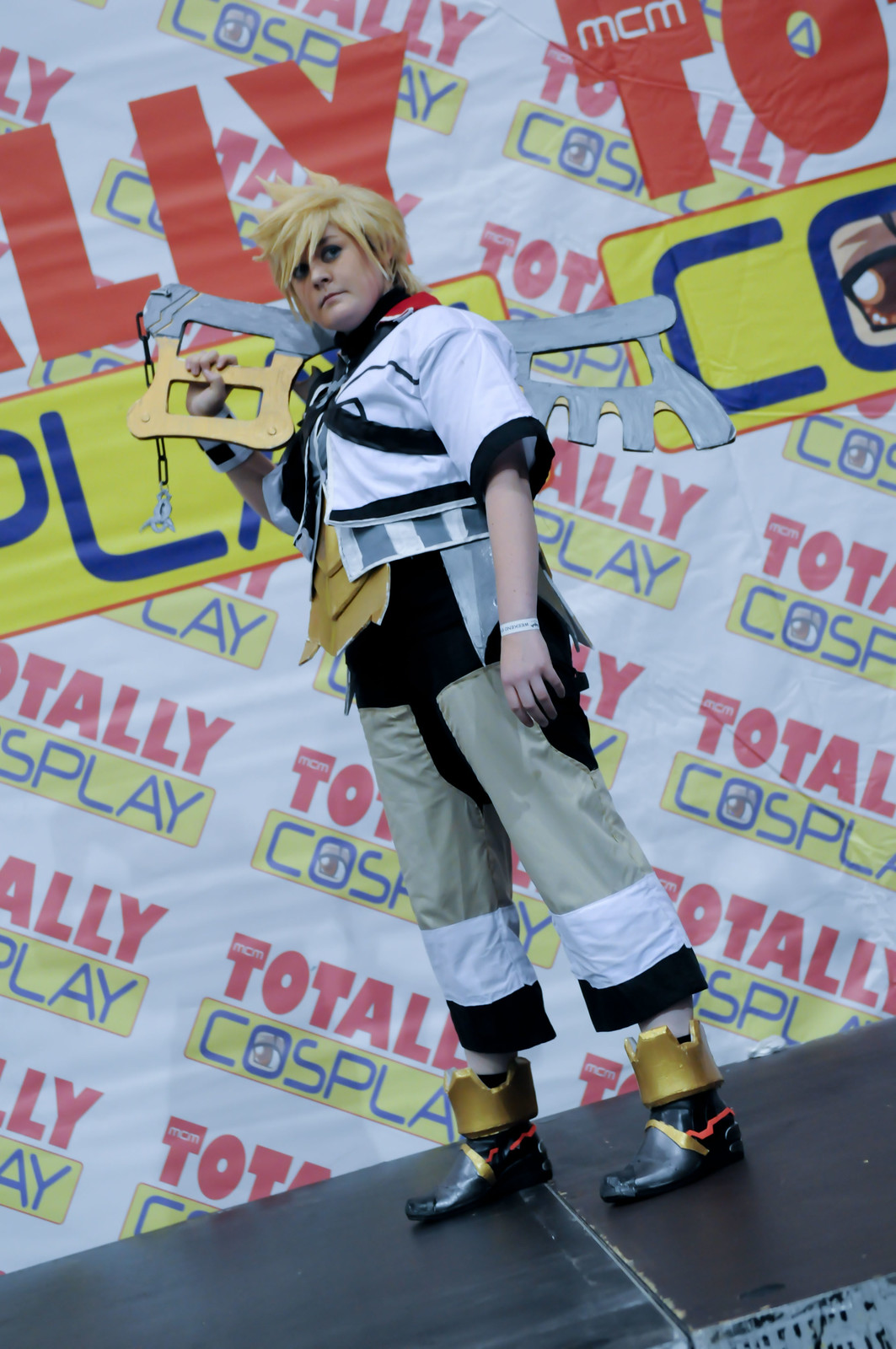The image captures an indoor cosplay event featuring a dynamic angle of a stage. Centered on the black stage is an individual in elaborate costume, likely a character from "Kingdom Hearts," identifiable by their handmade replica of a keyblade sword rested on their shoulder. The cosplayer, whose gender is indistinguishable due to the costume, sports styled spiky blonde hair, black and golden boots with red accents, multicolored trousers with shades of black, white, and grey, and a detailed top adorned in white, black, and golden hues alongside numerous belts. The backdrop features a prominent banner reading "Totally Cosplay" in bold, with "Totally" in red font and "Cosplay" within a yellow box with blue font. The setting suggests an exhilarating festival atmosphere.